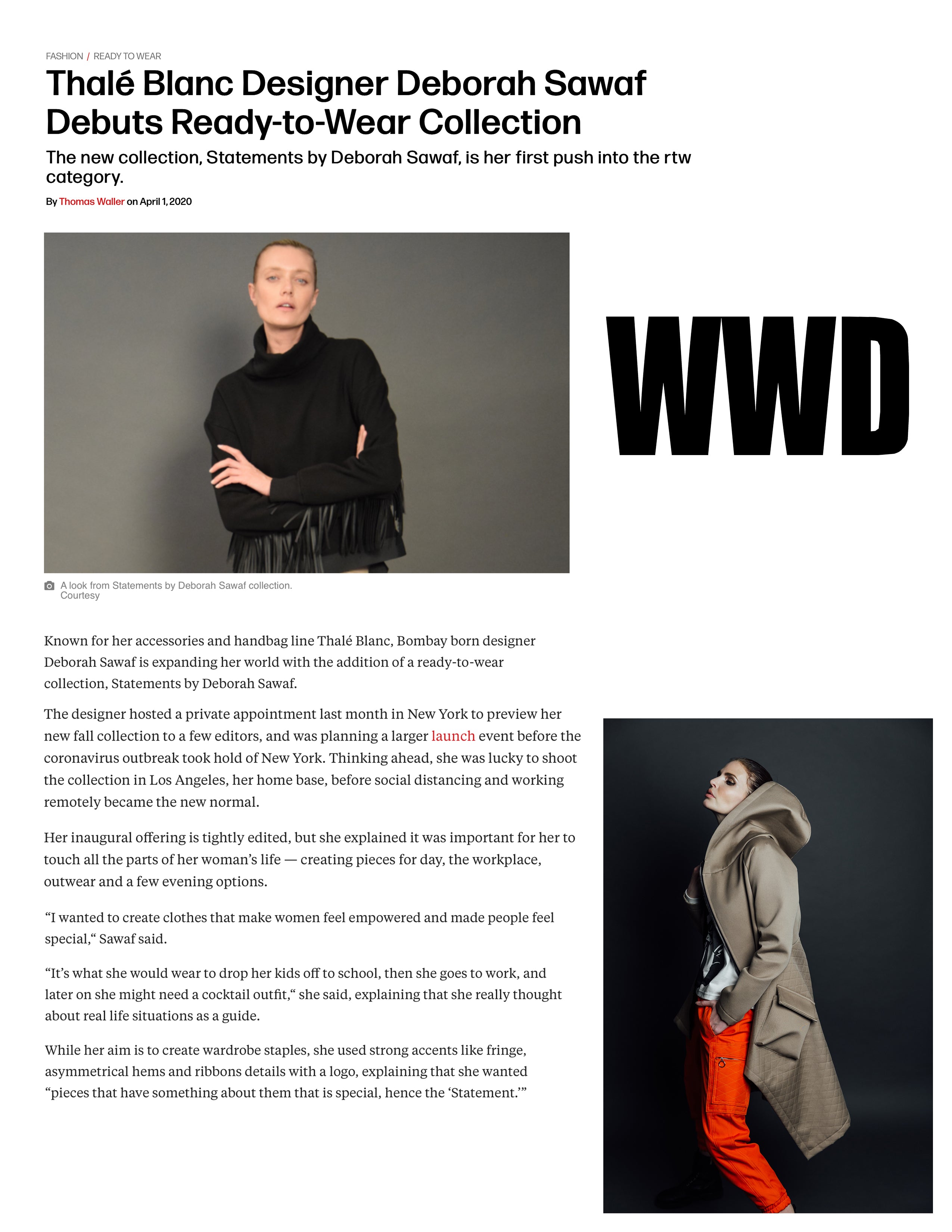This image is a screen capture of an article prominently featuring Thalé Blanc designer Deborah Savoieff, with a headline that reads "Thalé Blanc designer Deborah Savoieff debuts ready-to-wear collection." The subheadline elaborates that the new collection, Statements by Deborah Savoieff, is her first foray into the ready-to-wear category. Written by Thomas Walker and dated April 1st, 2020, the article contains six paragraphs detailing the collection along with quotes from Savoieff herself. A "WWD" logo is visible, potentially indicating the source of the article.

The image highlights two distinct photographs. In the foreground, there is a picture of Deborah Savoieff dressed in a black ensemble, with her slicked-back hair exuding a sleek and modern look. Right below the headline, we see a detailed portrait of a model dressed in a black turtleneck sweater paired with what appears to be a leather pleated skirt, accessorized with a handbag tucked under her arm. Her arms are crossed in the photo, and her short hair frames her face as she looks forward. 

Additionally, another photograph showcases a different female model, possibly from the same collection, standing in profile. This model is dressed in a beige overcoat, orange pants with pockets, and a white shirt. She has her left hand in one of the pockets, looks upwards, and, like Savoieff, her hair is slicked back to complement the modern and chic appearance of the collection.